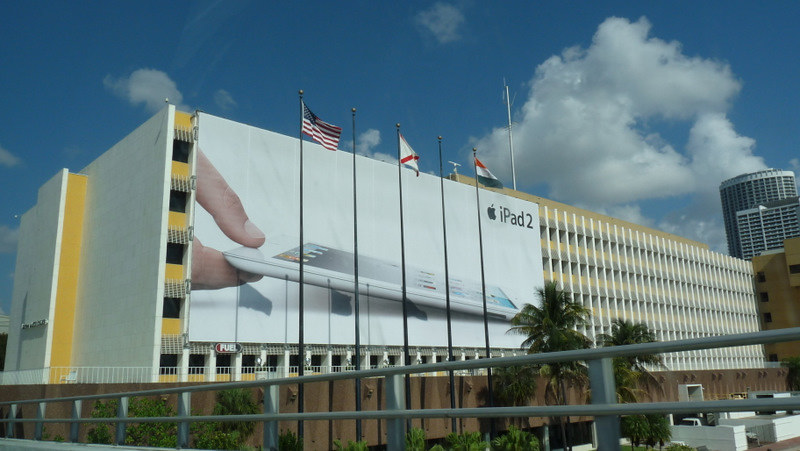An elevated photograph captures a bird's-eye view over a gray fence or guard rail, revealing a parking lot below. A sprawling structure dominates the scene, stretching diagonally from left to right and appearing more massive on the left. The five or six-story industrial building sports a white exterior with yellow highlights and numerous dark cubicles, indicative of an open-sided parking garage. 

A striking feature is the large white billboard plastered across the left half of the building's front, depicting an iPad 2 held between someone's index finger and thumb, tilted downward onto a table. The upper right corner of the billboard displays the text "iPad 2" alongside an Apple logo. The building's base transitions into a red or sandstone brown hue, with visible cement barricades and the tops of cars in the lower right corner. An extension of the red sandstone brick runs up the right side of the image, joining the white building to a towering, slightly leaning circular gray structure in the background. 

The sky above is a clear blue adorned with white clouds. In front of the iPad billboard stand five flagpoles, the leftmost bearing a clearly visible American flag, while the flags on the other poles are indistinguishable.